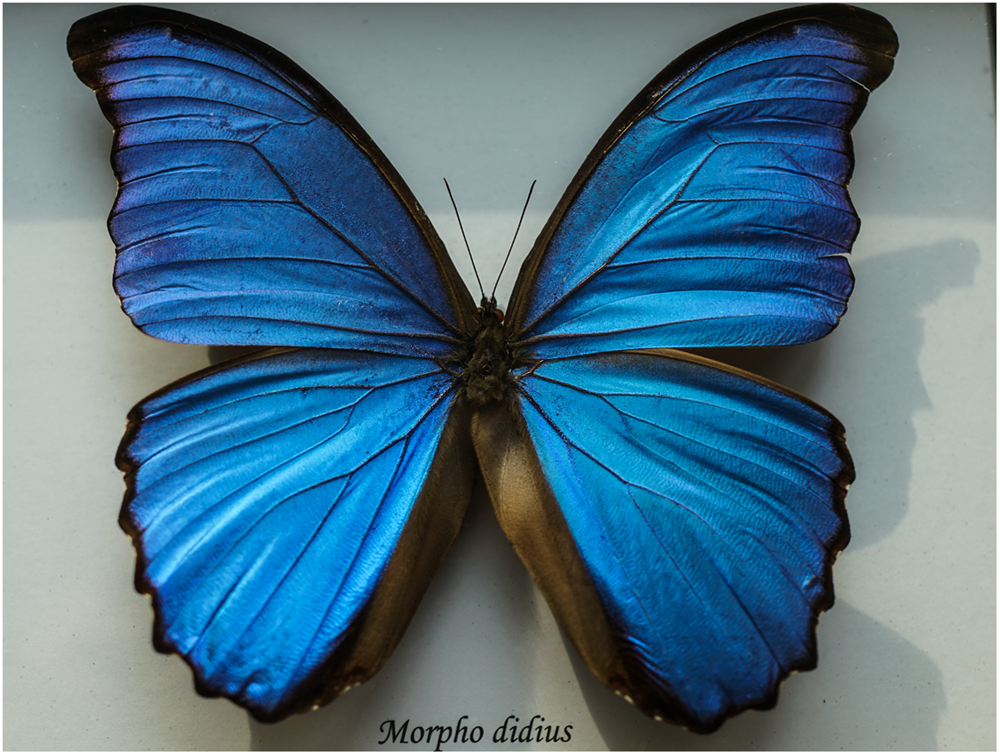The image is a close-up photograph of a large blue butterfly, possibly an art piece or a preserved specimen, set against a light gray, featureless background that casts shadows to the right. The butterfly's vibrant blue wings dominate the frame, with the tops of the wings touching the top edge and the bottoms nearly reaching the bottom edge. The wings are a vivid aqua blue with intricate, rippled variations in shading, edged by black veins and borders that transition into a subtle brown. The butterfly's body is black, slightly dried and rolled in appearance, with a small, black head and long, thin, black antennae extending from it. The text "Morpho Didius" is written in black italic font at the bottom of the photograph.